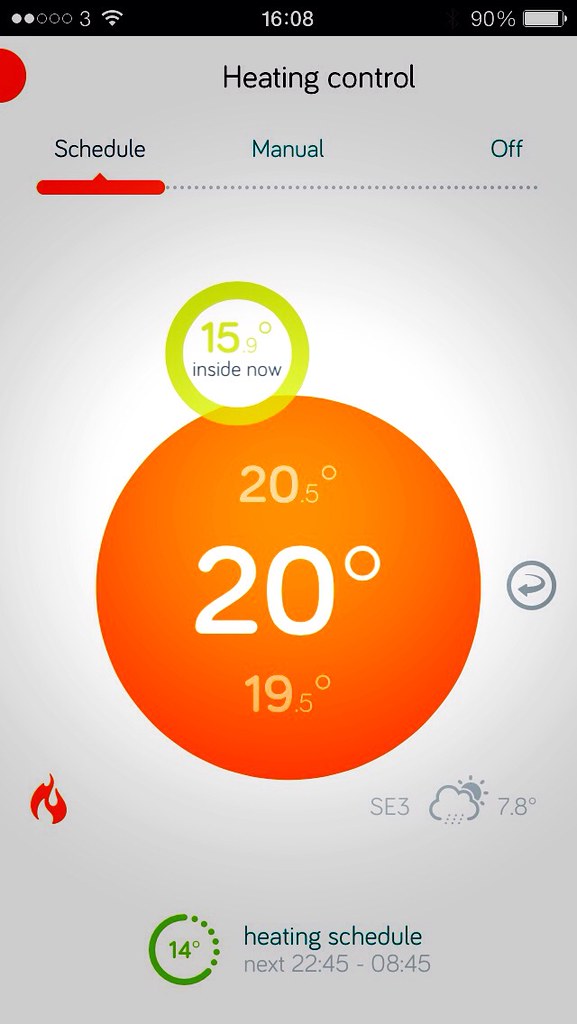The image depicts a white digital display panel that monitors and controls the heating system. At the top of the display, the time is clearly shown as "16:08," with a Wi-Fi symbol on the left and a battery icon on the right, indicating a 90% charge. Just below the time, the header reads "Heating Control" in black letters.

Directly beneath this header, the panel features three setting options: "Schedule," "Manual," and "Off." Central to the display is a prominent large orange circle indicating the current set temperature of "20°C." Surrounding this main reading, smaller markings denote "19.5°C" below it and "20.5°C" above.

In the middle of the screen, a smaller yellow circle indicates the current indoor temperature as "15°C." Positioned under the orange circle, a symbol combines a cloud and sun, suggesting the weather is partly cloudy.

At the bottom of the display, the words "Heating Schedule" are displayed. Underneath, a small green marker indicates a temperature of "14°C" with a time interval noted as "22:45 - 08:45," signifying the scheduled period for this temperature setting.